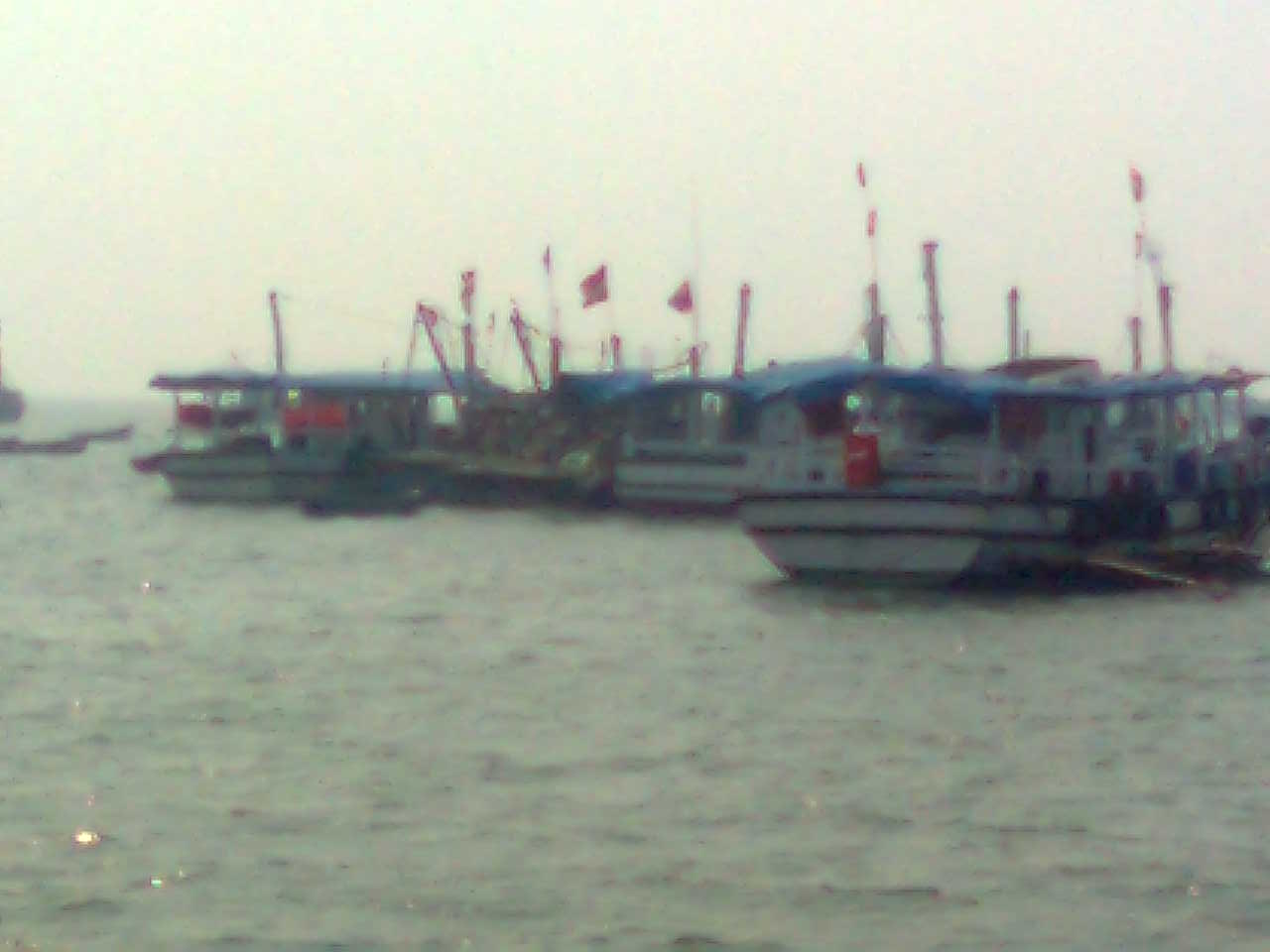A digital photograph captures a dock scene with a cluster of boats on the water, extending from the left center to the right center of the image. The picture is very blurry and somewhat out of focus, making details subtle. The water appears dark with calm ripples and no white caps. The sky above is a hazy, flat white, nearly blending with the water at the horizon. The boats are mostly white with crosswise stripes and have blue tarp roofs, likely offering shelter beneath them. These boats, arranged stern-first, bear poles with flags, predominantly in red, possibly resembling the Norwegian flag. Smaller boats and kayaks are also visible to the left. There are no people present, and a few poles, possibly indicating the pier connections, are faintly seen amidst the boats.